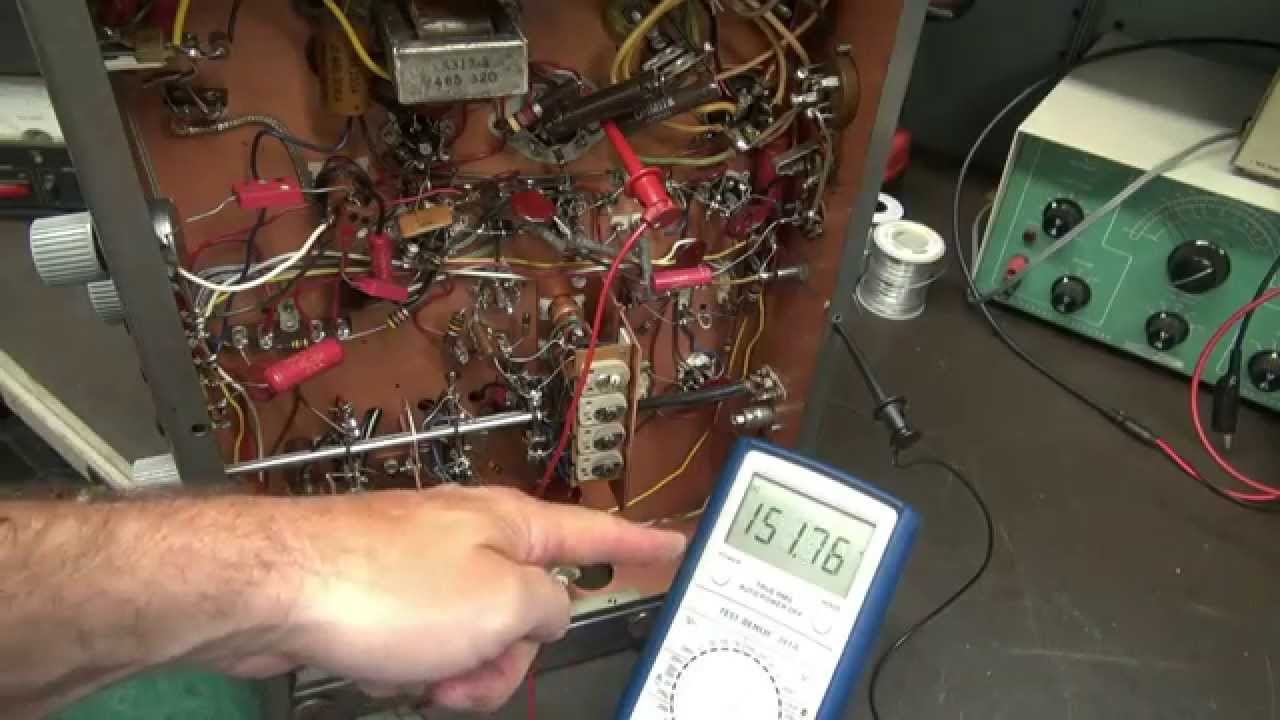In this detailed color photograph, a complex electronic contraption with its side panel removed reveals an intricate array of tangled wires and various components. At the center, a Caucasian man, identifiable by his very hairy hand, points while holding a digital multimeter displaying "151.76." To the right of the contraption, a teal-colored instrument with multiple black dials and knobs is visible, accompanied by red and black wires. Spools of metal wire, likely solder, and additional equipment rest on a brown tabletop, contributing to the scene of what appears to be an electronics workshop. The overall chaotic yet detailed setup speaks to the intricacies of electronic diagnostics and repair.